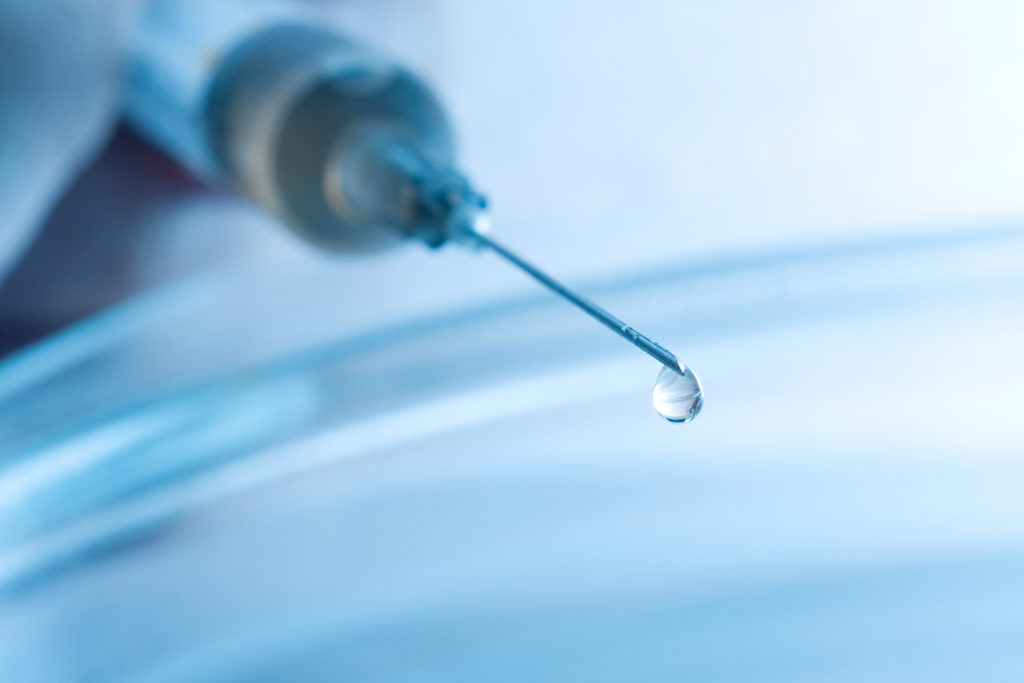The image is a high-definition, close-up photograph of a syringe dispensing a drop of liquid, captured with great clarity by a skilled photographer. The syringe is oriented from the upper left to the lower right, with the needle pointing towards the lower right. A single drop of liquid is poised at the needle’s tip, ready to fall. The main focal point is the elongated needle with the liquid drop, which stands out sharply against a blurred background. 

The surrounding environment features shades of blue and white, with a hint of a glass beaker or bowl positioned beneath where the drop might fall, suggesting precise, delicate control in the dispensing process. The syringe itself, along with any hand holding it, is blurred, drawing attention specifically to the needle and drop. The entire scene is suffused with light from the upper right, illuminating the drop and creating a contrast with the softer, out-of-focus elements and a subtle reflective surface underneath, likely a glass sheet or container.